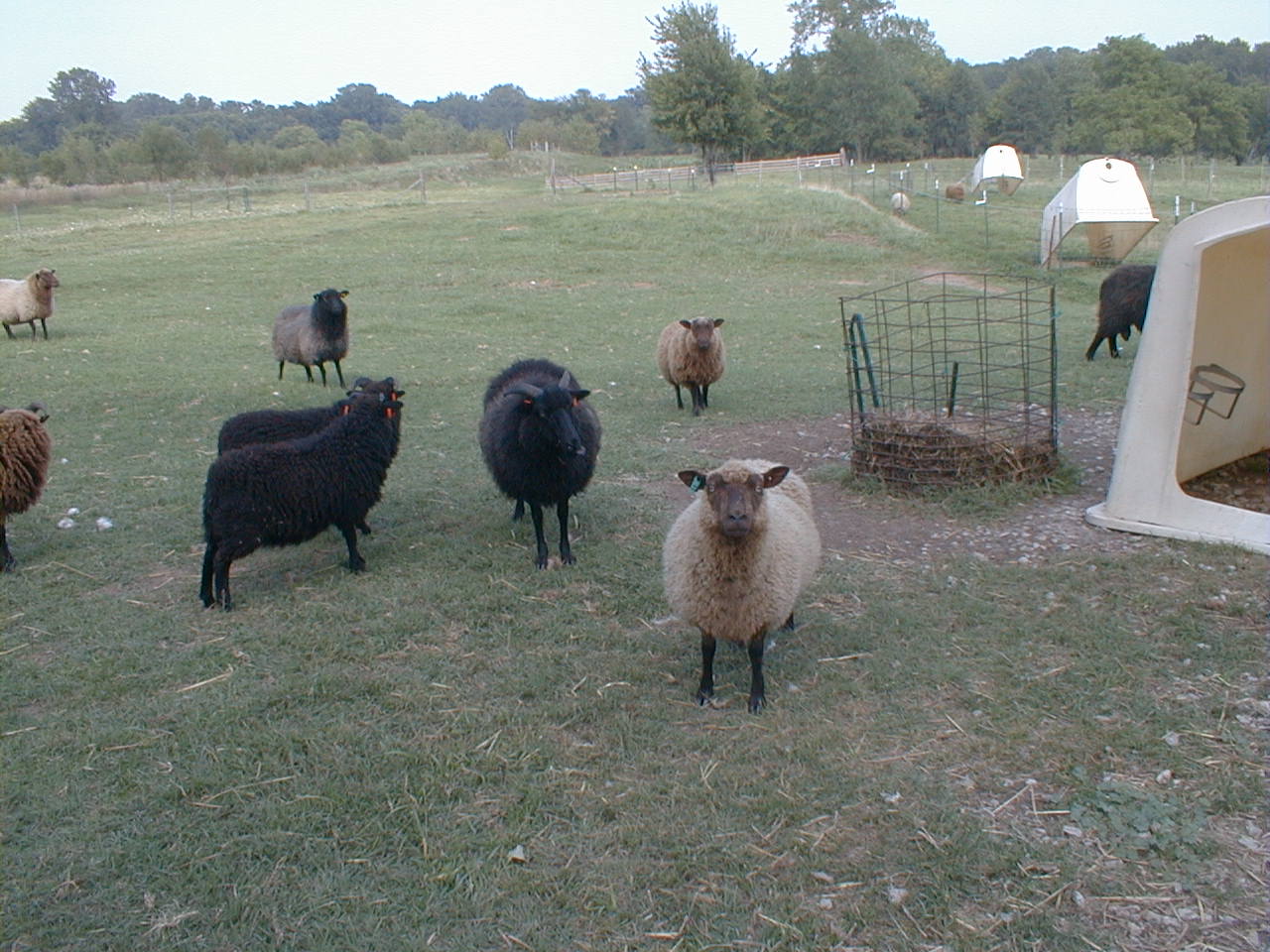The image depicts a bucolic farm scene with a meadow in the foreground and a dense forest on the horizon beneath a light blue sky. A variety of structures dot the pasture, including three igloo-style plastic shelters, some of which are propped up—likely to encourage the sheep to graze and exercise, keeping them out during the day. The area is enclosed with a combination of wooden picket fences and chain-link wire fencing. 

In the meadow, there are eleven sheep of various colors and sizes. The sheep closest to the camera is an off-white with a brown snout and black legs, looking directly at the camera. There are three black sheep nearby with black legs, ears, and horns, each tagged with an orange marker on their ears. Further back, a gray sheep with a black head and legs stands next to a light brown sheep with a brown head. There are also tan sheep with black legs and a couple more off-white or tan sheep in the distance. One of the sheep in the middle of the image is a striking brown and black.

Additionally, several feeding structures are present, including a cage-like wired bin with hay inside, designed to provide dry feeding material for the sheep. The grass in the area is predominantly green but mingled with patches of brown straw, indicating a well-trodden pasture area. The background reveals a dense tree line, further emphasizing the serene, pastoral setting of the farm.